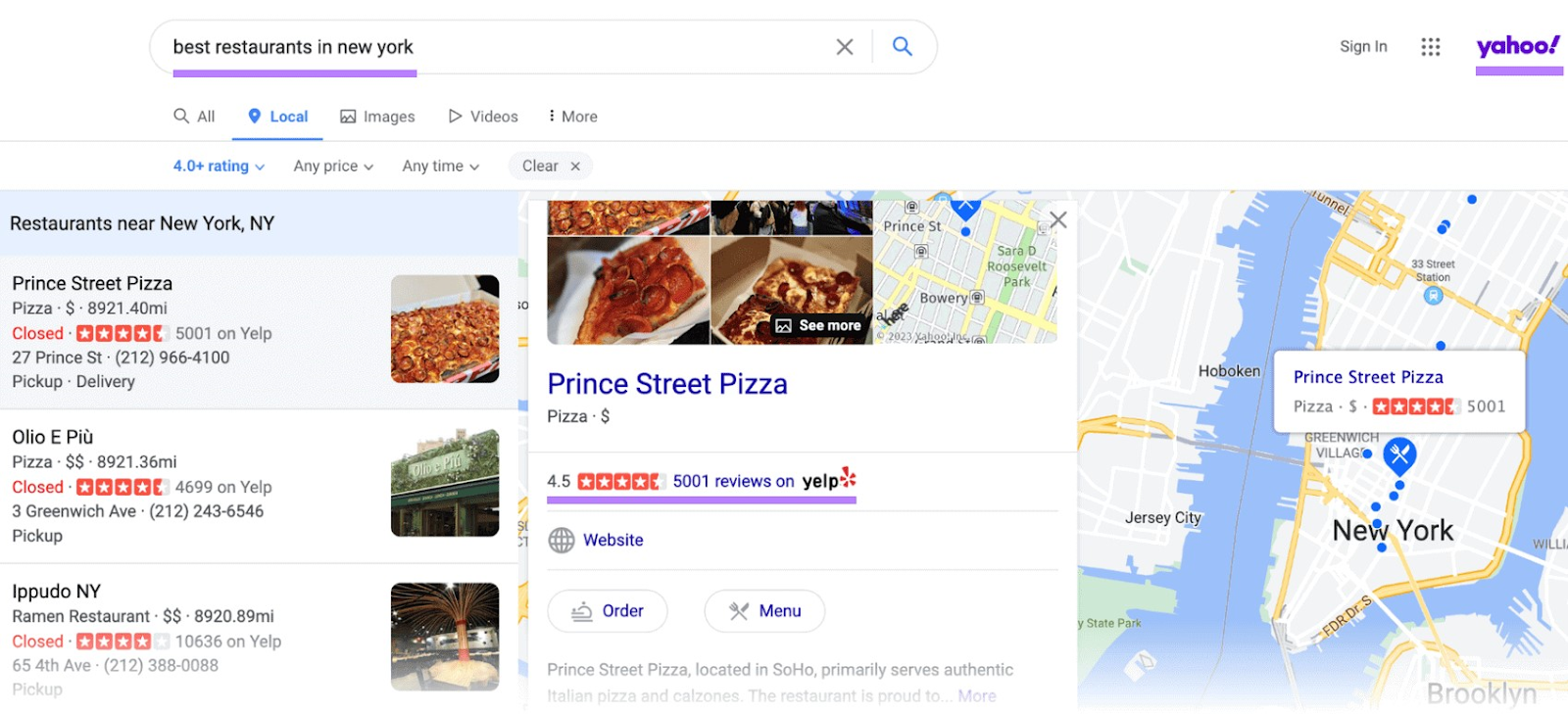The image displays a web browser with the search bar reading "best restaurants in New York." The search results show several restaurant listings near New York. The first result is "Prince Street Pizza," identified as a pizza restaurant, which is currently closed. The listing includes its address. Following that, "Olio e Pio" appears next, and then "Ippudo," which is described as a ramen restaurant. The page provides addresses and descriptions for each restaurant, helping viewers identify the type of cuisine and the operational status of the establishments.